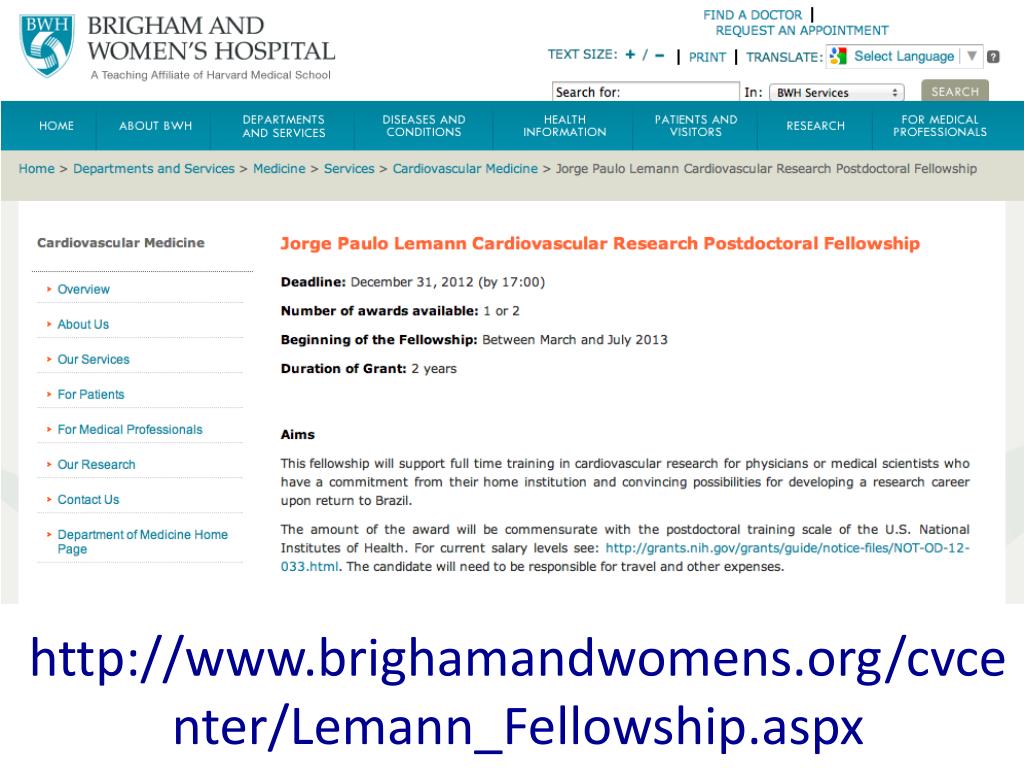The website homepage for Brigham and Women's Hospital features a prominent emblem shaped like a shield with the initials "BWH" displayed in blue. Across the top, a blue navigation band includes links labeled: Home, About BWH, Departments and Services, Diseases and Conditions, Health Information, Patients and Visitors, Research, and For Medical Professionals. Additionally, options to "Find a Doctor" and "Request an Appointment" are available at the top of the page, along with language selection and a search function.

The main content area features a grey-shaded sidebar on the left and a large white content box occupying the central space. Within this box, an announcement is highlighted in orange about the "George Paulo Lehman Cardiovascular Research Postdoctoral Fellowship." Key details include:

- Application deadline: December 31st, 2012 by 17:00
- Number of awards available: 1 or 2
- Fellowship start date: Between March and July of 2013
- Duration of the grant: 2 years

The fellowship aims to support full-time training in cardiovascular research for physicians or medical scientists with a commitment from their home institutions in Brazil, and with clear potential for developing a research career upon their return.

The grey-shaded sidebar on the left includes links to various sections: Overview, About Us, Our Services, For Patients, For Medical Professionals, Our Research, Contact Us, and Department of Medicine Homepage. The URL for the website is prominently displayed in large purple letters at the bottom of the page.